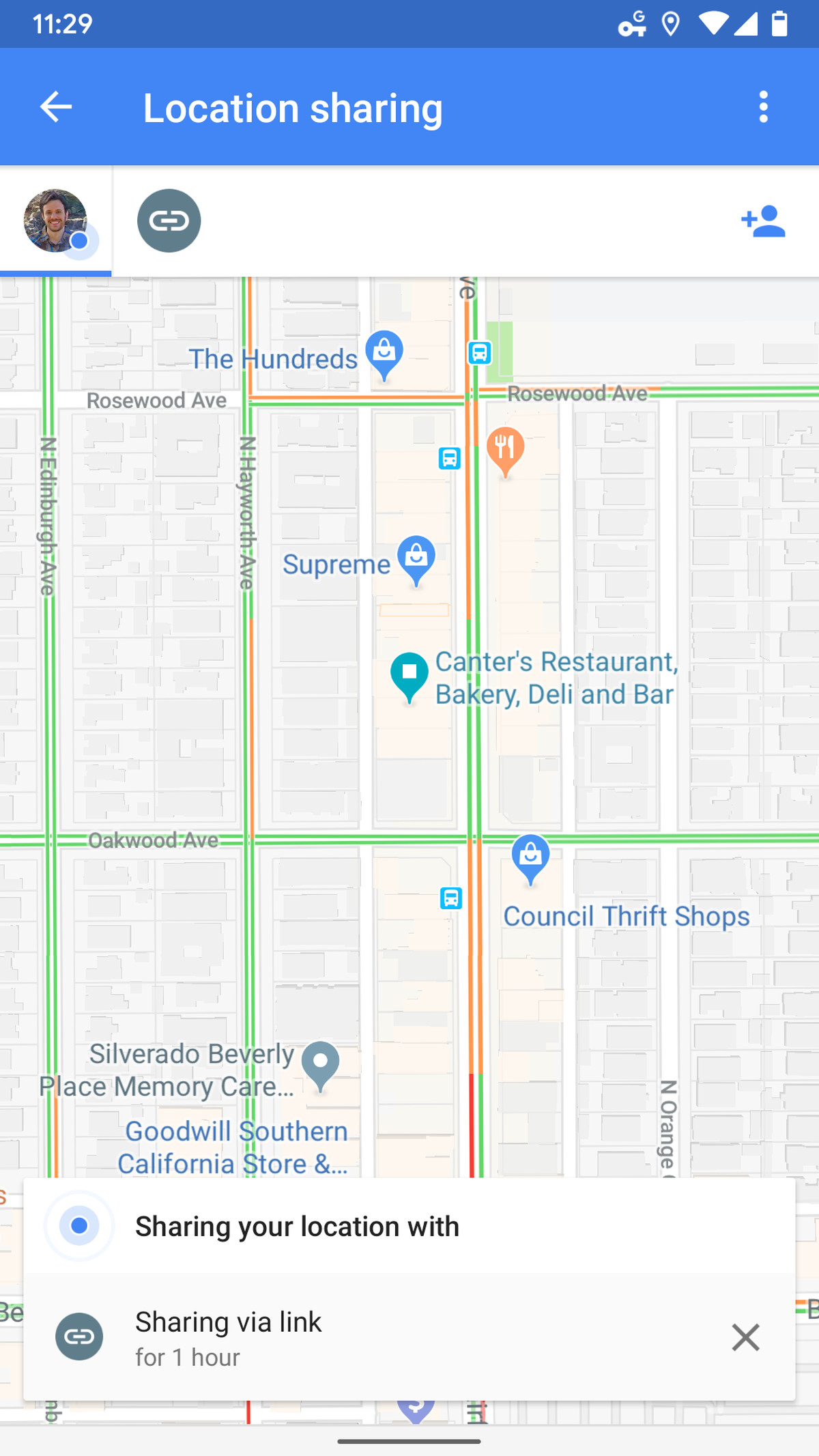The image depicts a screenshot of a map from a mobile phone. At the top of the screenshot is a blue navigation bar with a white arrow pointing to the left, followed by the text "Location sharing." Just below this navigation bar is another white bar which contains a small, round profile photo, a chain link icon, and a blue icon of a person with a plus sign, indicating options for managing location sharing.

The main portion of the screenshot shows a standard Google map with a grid of streets. The map features two prominent streets running vertically and three streets running horizontally. Notable landmarks and businesses marked on the map include the Council Thrift Store, Silverado, Beverly Place Memory Cafe, Goodwill Southern California Store, Canner's Restaurant, Bakery, Deli and Bar, Supreme, and The Hundreds. The streets on the map are highlighted in green, typical of Google Maps, providing clear visual guidance to the viewer.

In summary, the image provides a snapshot of a location-sharing screen with a detailed view of a specific area, highlighting various points of interest and showcasing the map's intuitive design.